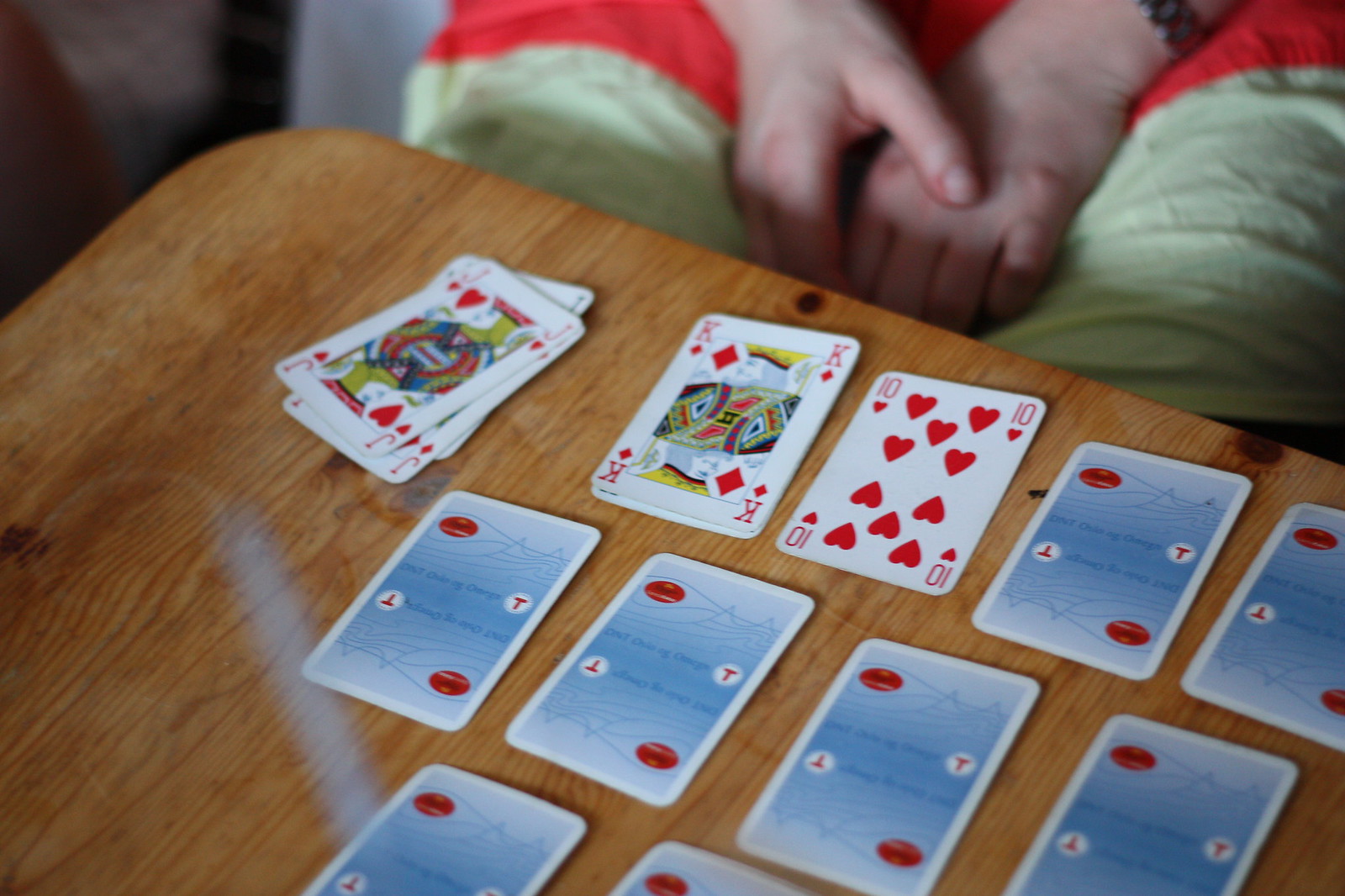From my vantage point, the image depicts a person seated at a wooden table in good condition, its brown surface showing some characteristic spots. The individual is not fully visible; only their hands resting in their lap can be seen, which appear child-like. They are dressed in green and red pants. In front of them lies an array of playing cards. Some cards are face down, including two in the top row, four in the second row, and two on the left in the third row, concealing their identities. On the bottom row to the right, there is a stack of cards, while next to this stack, the visible cards include a ten of hearts and a king of diamonds, which seems to be placed atop another card. The background in the upper left corner features an indistinct white space, possibly part of the wall or furniture trim near where the child is playing.